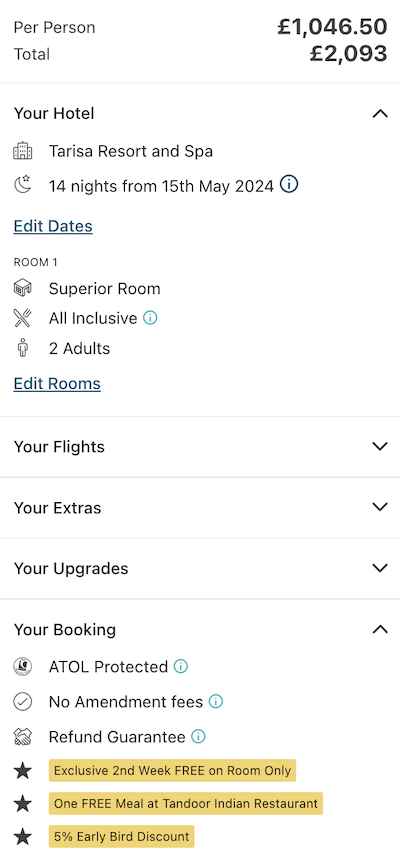The image depicts a detailed breakdown of a bill, possibly related to a vacation package. The background is white with key information prominently displayed. At the top, the phrase "Per Person" is visible, which is followed by an amount of £1,046.50. Below this, the total sum of £2,093 is displayed, separated by a line.

Next, the details regarding accommodation are provided. An icon of a hotel precedes the text "Teresa Resort and Spa," accompanied by a crescent moon symbol. To the right, it specifies "14 nights from 15th May 2024" with an option to "Edit Dates" in a blue link. Listed further are room details with another building icon, mentioning "Room 1." It describes the accommodation as a "Superior Room" with a fork and knife icon and "All Inclusive" indicated, accompanied by an informational icon. The text "Two Adults" appears next, preceded by a person icon, and there is an option to "Edit Rooms."

Separators delineate different sections of the bill. Following the accommodation details are sections titled "Flights," "Extras," and "Upgrades," each with a dropdown arrow to the right for further details. Another line separator follows, leading into the "Booking" section.

Under "Booking," there is a "TOL Protected" icon followed by a shield symbol, "No Amendment Fees" with a check mark icon, and "Refund Guarantee" with a handshake icon. Each of these features is accompanied by a circular information icon centered with the letter "i."

Beneath these features are three highlighted incentives, each marked with a star icon. They read: "Exclusive Second Week Free on Room Only," "One Free Meal at Tandoor Indian Restaurant," and "5% Early Bird Discount," all highlighted in yellow.